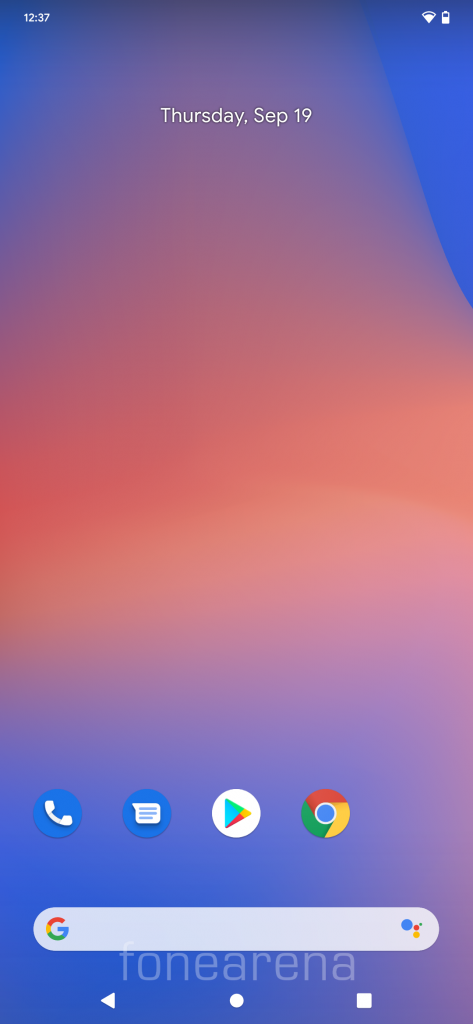The image displays a screenshot from a cell phone. The background is a gradient of dark blue blending into bands of purple and pink hues. In the upper-left corner, the time "12:37" is displayed in white. Centrally positioned is the date, "Thursday, September 19th." On the upper-right corner, icons for a nearly full Wi-Fi signal and a battery at 75% capacity are visible.

At the bottom portion of the screen, several app icons are aligned:
1. The Phone app: Represented by a dark blue circle containing an icon of an old-fashioned landline phone in white.
2. The Samsung Chat app: Depicted by a dark blue circle featuring a white chat bubble with cyan blue accent lines.
3. The Google Play Store app: Illustrated by a white circle with an overlaid multicolored triangle, showcasing blue at the bottom, green on the right, yellow transitioning into red.
4. The Gmail app: Comprised of four colored quadrants—green, red, yellow, and dark blue—with a white border.
5. The Google app: Displayed as a dark gray oval-shaped rectangle with a multicolored "G" on the left (painted in red, orange, green, and blue) and a series of small circles (dark blue, red, orange, green) on the right.

Below these icons, the text "PHONEARENA" appears twice in gray.

On the bezel of the phone, navigation icons including a triangle, a square, and a circle are presented in bold white.